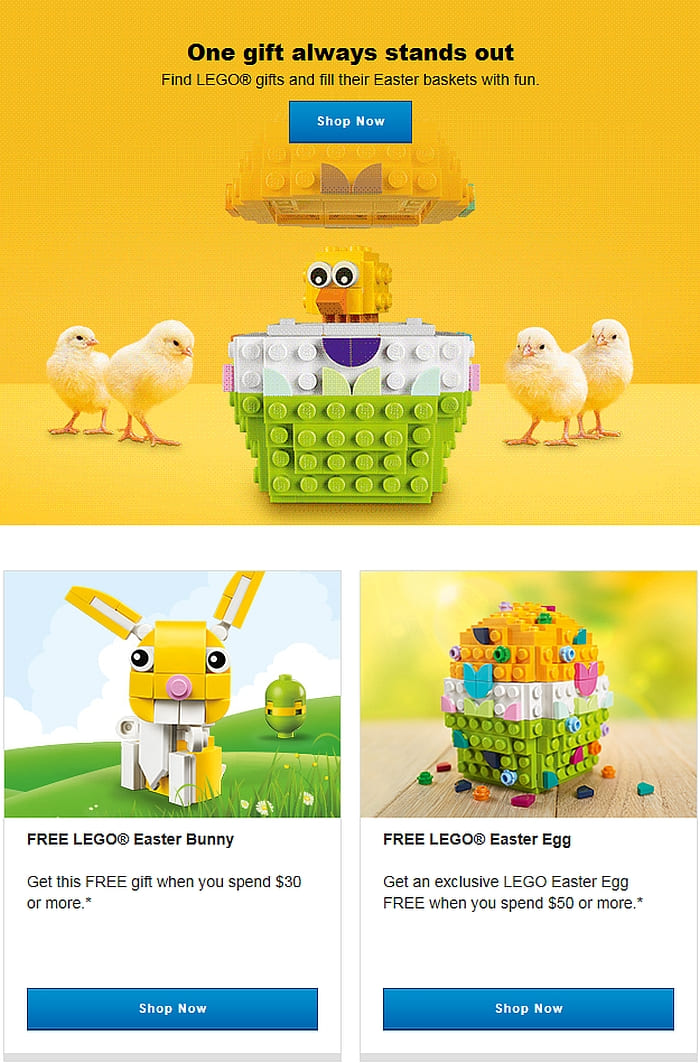The image is divided into three sections. 

### Top Section:
The background features a gradient of yellow shades, creating an ombre effect. At the center, in bold black text, it reads: 
"One gift always stands out. Find Lego gifts and fill their Easter basket with fun." 

Above this text, there are yellow Lego bricks. Below the text, a blue rectangle with the text "Shop Now" in white sits between two sets of two chicks, making a total of four chicks surrounding the message.

### Middle Section:
This section showcases a Lego creation of a colorful chick. The chick has a green body, white wings, a purple belly, and a yellow head with distinct eyes and a beak. To the left, there is a Lego bunny with a yellow and white construct, a pink nose, and expressive eyes. It stands on a patch of green Lego grass with white Lego flowers.

Next to it, there is another Lego structure, possibly a Lego egg, composed of green and yellow bricks. The sky backdrop is blue with white clouds.

### Bottom Section:
Here, in clear black text, it states: 
"Free Lego Easter Bunny! Get this free gift when you spend $30 or more." 
Below this message, there is another blue rectangle with "Shop Now" written in white.

Further down, it states: 
"Free Lego Easter Egg! Get an exclusive Lego Easter egg free when you spend $50 or more." This message includes an asterisk indicating additional terms. Additionally, this section features another blue rectangle with the text "Shop Now."

The section concludes with an array of stacked Lego bricks in various colors, including green, white, yellow, pink, blue, and purple, arranged randomly near the bottom edge of the image.